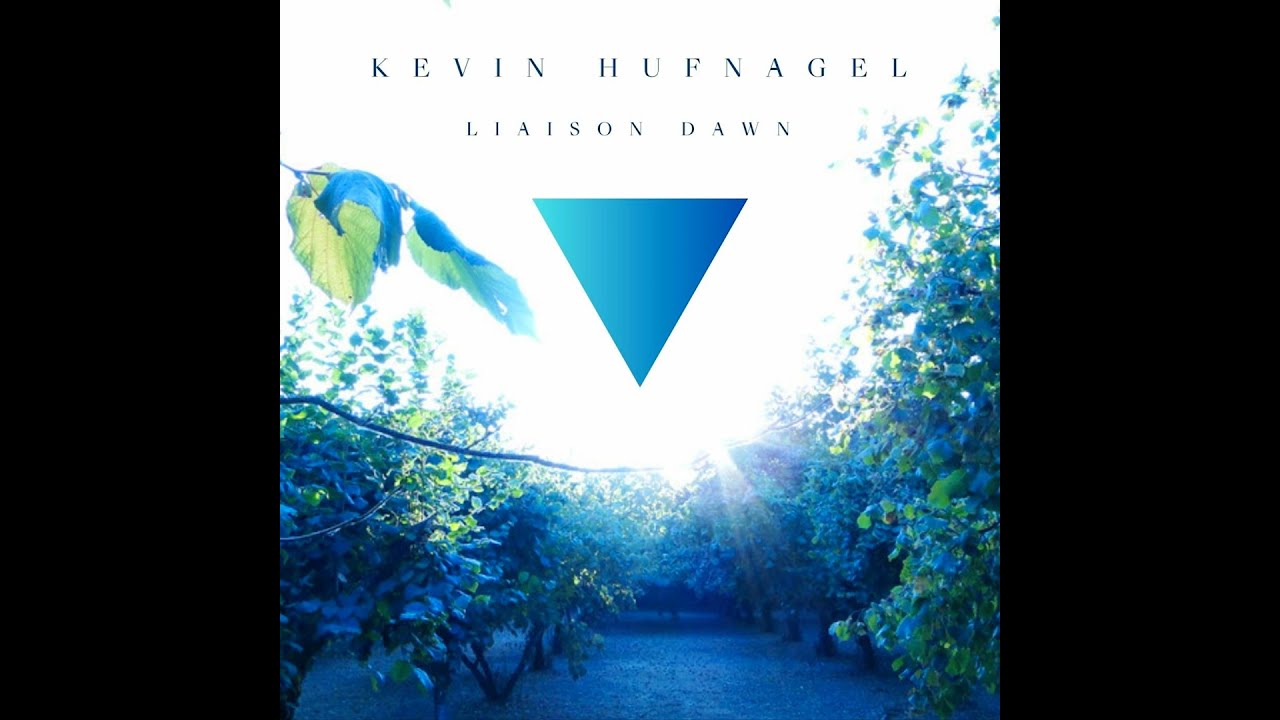This image appears to be the cover of an album, featuring the name "Kevin Hufnagel" in capitalized letters at the top, followed by "Liason Dawn" just below it, also in capitalized letters. Both lines of text are floating at the top of the image against a blinding white sky, accented by rays of light. Below the text, there is a striking blue equilateral triangle, inverted with its point facing downward, transitioning from dark to light blue.

The artwork captures a scenic farm or garden, predominantly tinted in blue and green hues. The scene reveals an orchard with a pathway lined by trees, with lush green leaves. The camera perspective is elevated to human height, offering a clear view down the pathway. Black vertical bars frame the sides of the image, emphasizing the square central artwork. The combination of natural elements and ethereal lighting creates a serene yet mysterious atmosphere.